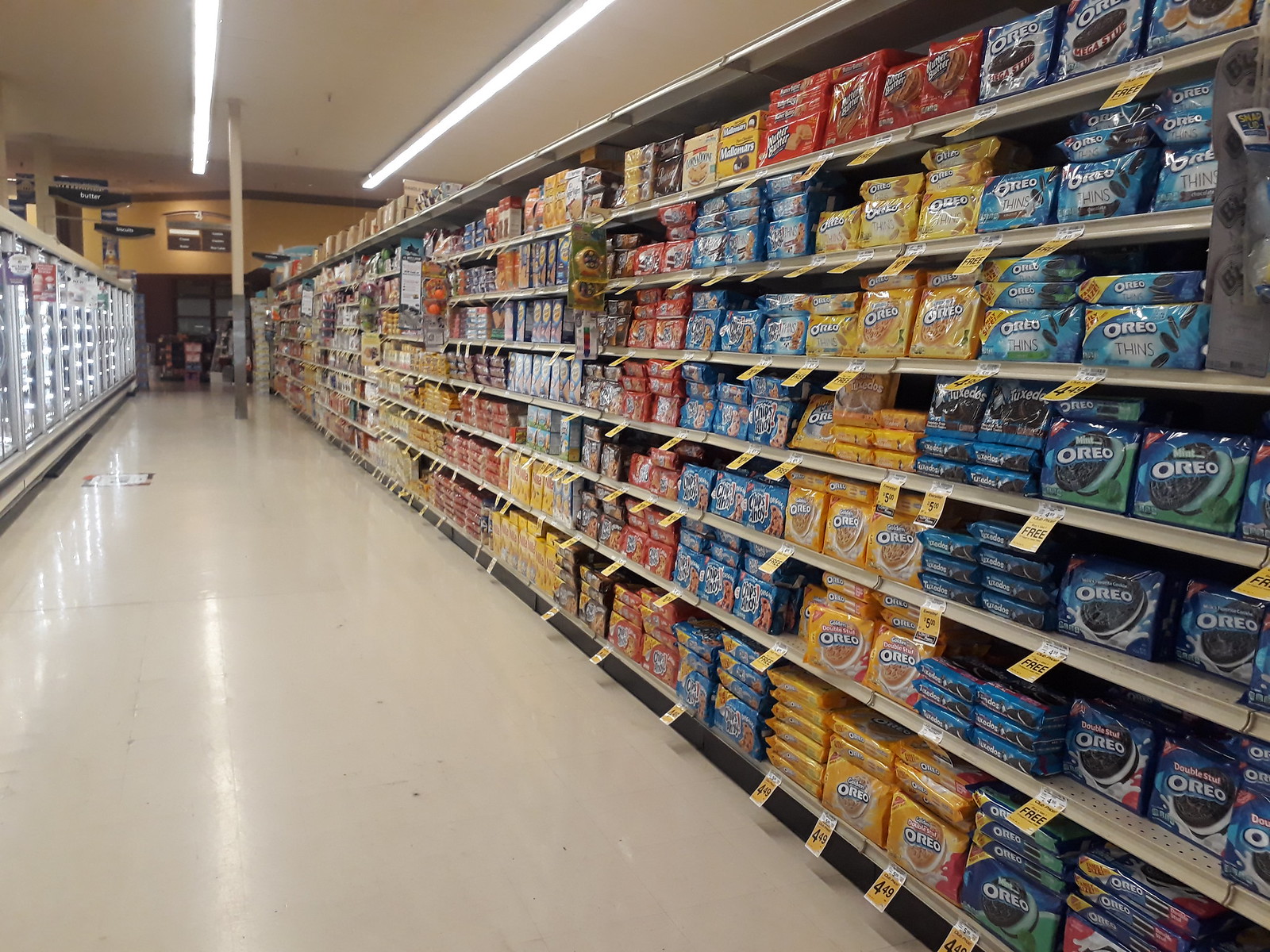This vibrant photograph captures the bustling cookie aisle of a grocery store. The aisle, showcasing an impressive seven levels of cookies, runs the length of the image. On the left, a refrigerated section glows faintly, its contents indistinguishable from this distance. Directly ahead, a beige-colored support beam wrapped in gray stands before a set of windows that could be part of a managerial office. Overhead signs denote various aisle sections including a faintly visible "butter" sign towards the frozen area.

The cookie aisle is a colorful panorama filled with various brands and types. Prominent among the selections are several varieties of Oreos, including Mega Stuff, Thins, Mint, Golden, Double Stuffed, and Tuxedo Oreos. Further down the aisle, different types of Chips Ahoy! line the shelves, available in red and blue bags, along with Nutter Butter cookies in red packaging. Also visible are boxes of Cheez Whiz, yellow and blue, alongside other colorfully packaged snacks. Clear price tags and promotional stickers, like "buy one, get one free" and prices like $4.49, are prominently displayed.

Illuminating the perspective, lights affixed to the ceiling highlight the smooth white floor, providing a clear, easy-to-navigate passage for shoppers. The combination of vibrant packaging, well-organized shelves, and strategic lighting makes this grocery store aisle an inviting haven for snack enthusiasts.